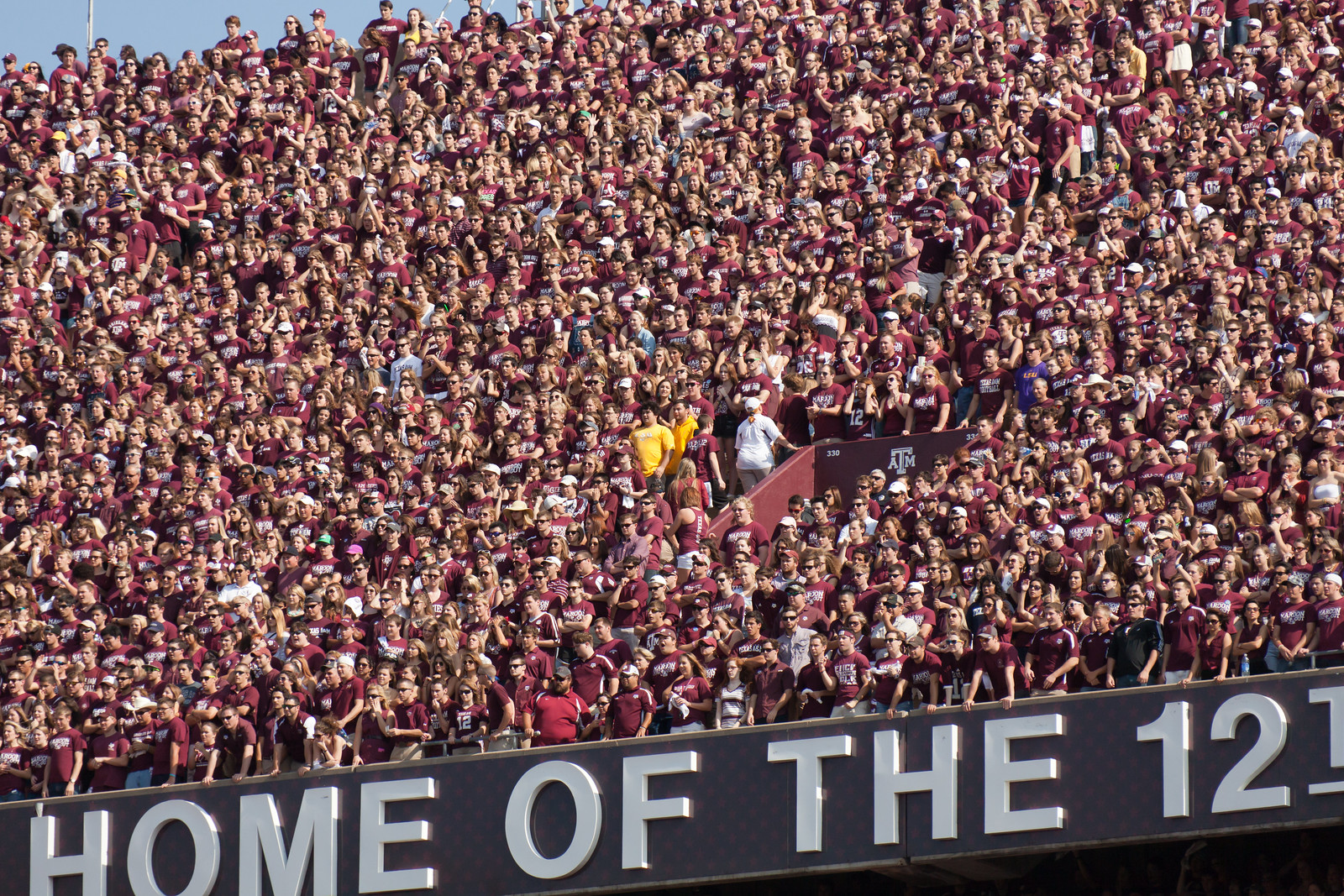The photograph captures a vibrant outdoor scene during a sporting event, set on a bright, sunny day. The image focuses on a large crowd of spectators, predominantly dressed in dark maroon shirts, filling the upper level of a stadium’s bleachers. In this sea of maroon, two individuals in bright yellow shirts notably stand out. Additionally, a woman in a white hat and white t-shirt is seen walking up the stairs, while a few other attendees sport white shirts and one person is wearing a navy shirt. The lower part of the image shows the underside of the bleachers cast in shadow, contrasting with the well-lit upper sections. A gray wall above the bottom right corner prominently displays the text "Home of the 12th" in bold white font. To the top left, a sliver of blue sky is visible, framing the energetic atmosphere. Spectators in sunglasses lean over the edge of the stadium, immersed in the event.